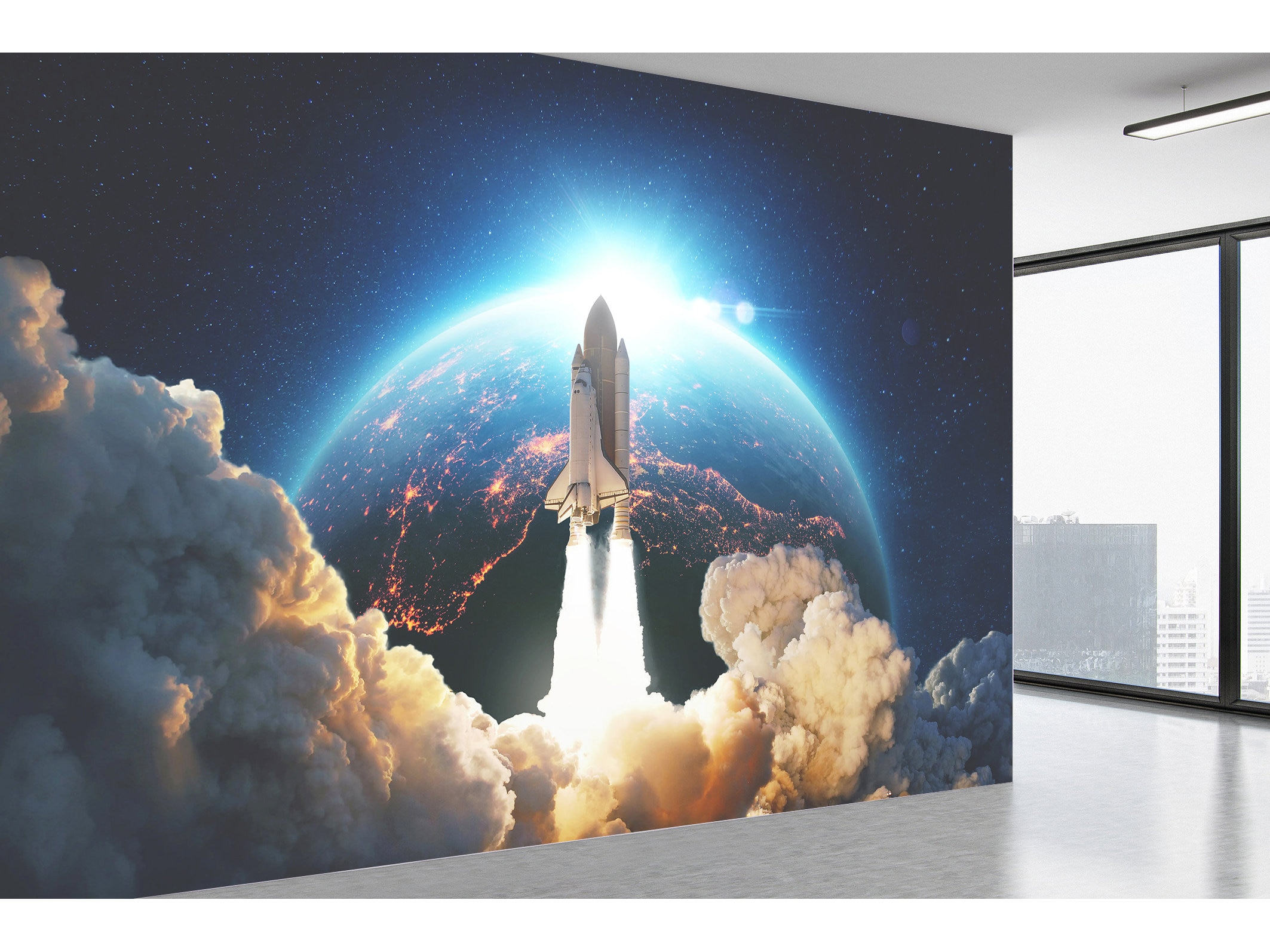The image showcases a detailed mural installation within a high-rise office space. The mural, located on the left side of the room, depicts a stunning space scene with a NASA spacecraft launching into the cosmos. The rocket is shown amidst a billowing plume of smoke, with Earth, captured in a nighttime perspective, dramatically hovering in the background. This creates an intriguing juxtaposition as the spacecraft appears to be taking off from within space itself. Surrounding the Earth are hyper-realistic clouds and twinkling stars, adding to the vivid celestial ambiance. The room features an off-white interior with a grayish floor, while large windows on the right reveal a hazy daytime sky and the tops of distant skyscrapers, accentuating the high-altitude setting of the office. This artwork may be a 3D-rendered piece, given its realistic yet slightly surreal elements.